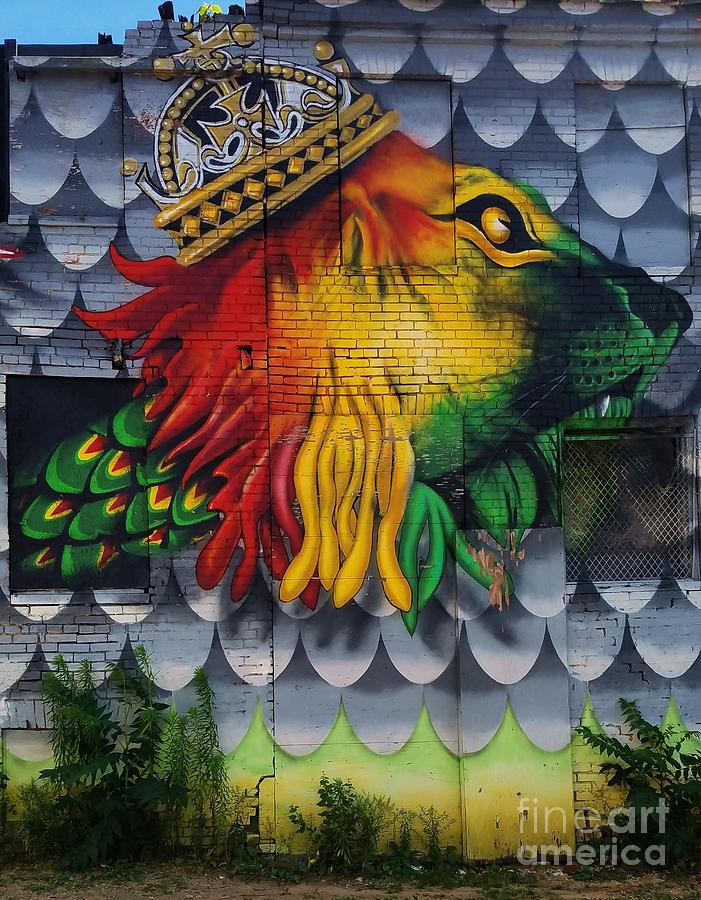The image captures an outdoor mural painted on a lavender-purple brick wall, partially visible due to a clear blue sky in the top left corner. At the bottom, there is a patch of brown dirt with shrubs and bushes growing against the wall. The very bottom of the mural features a layered pattern of stylized water waves transitioning from yellow to green, and then to light gray, medium gray, and dark gray. This wave pattern repeats upwards along the wall. The centerpiece of the mural is a striking depiction of a lion facing to the right, adorned with a golden crown that includes intricate, pointy designs, suggesting a regal or possibly religious connotation. The lion, composed of vibrant colors, showcases a green nose and neck, a yellow middle with one visible eye, and a red back of the head and mane. The lion's body appears to have green, light green, dark green, yellow, and red scales. Additionally, the mural contains white semicircles accents, and there's a painted section featuring blue petals. At the bottom right corner, the words "Fine Art America" are inscribed in white.